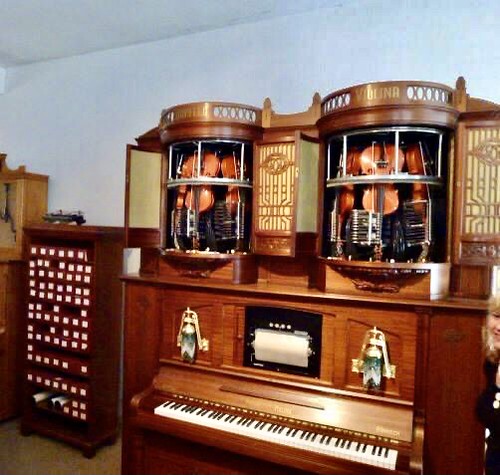In this image, we are inside a room with white walls, where an antique musical organ, crafted from rich cherry wood, prominently stands. The front of the organ reveals a set of black and white keys, reminiscent of a traditional piano, with a roll of paper situated above them, hinting at its player piano functionality. Above the keyboard, a series of curved, decorative glass windows adorn the instrument, behind which several violins are meticulously displayed. To the left of the organ, there is a matching cherry wood shelf, filled with numerous rolls of music paper intended for the organ’s automated performances. This shelf stands next to a taller wooden structure of a lighter brown shade, possibly containing drawers with white-fronted, box-like ends, adding further storage space to the room. Together, these elements create a nostalgic and elegant ambiance, giving the impression of a historic, well-maintained musical space.